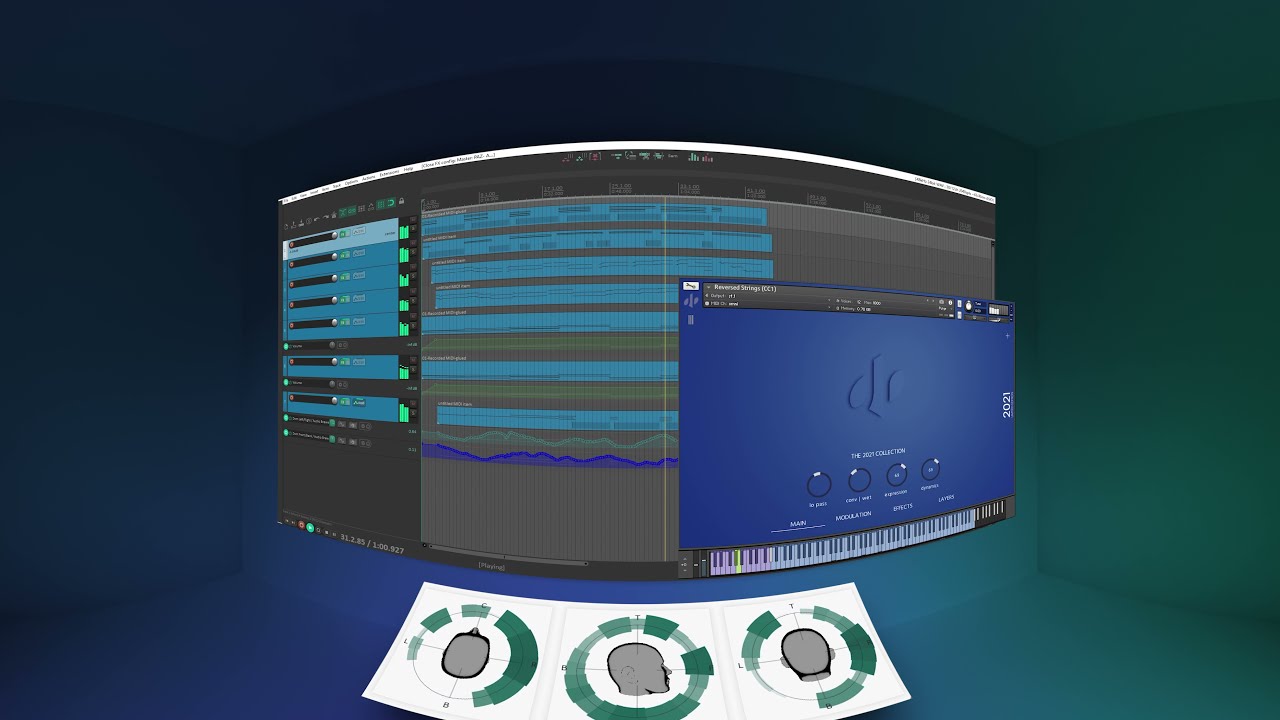The photograph showcases a detailed interface of audio editing software set against a gradient background transitioning from bluish on the left to a forest green on the right. Central to the image is a curved computer screen displaying various design elements typical of audio editing programs, including multiple wavy lines that seem to represent sound waves in shades of blue, green, gray, and black. The screen has seven prominent horizontal blue rectangles that mimic track layers with a mix of line graphs indicating sound levels or frequencies. Towards the bottom right, a black and white keyboard-like feature is visible. Below this main display, there's a white rectangle containing three green circles, each encapsulating the silhouette of a human head turned in different directions, encircled by green bars resembling sound levels or volume indicators. The overall scene gives a panoramic feel with a strong presence of vibrant symbols and graphical data points too minute to decipher.